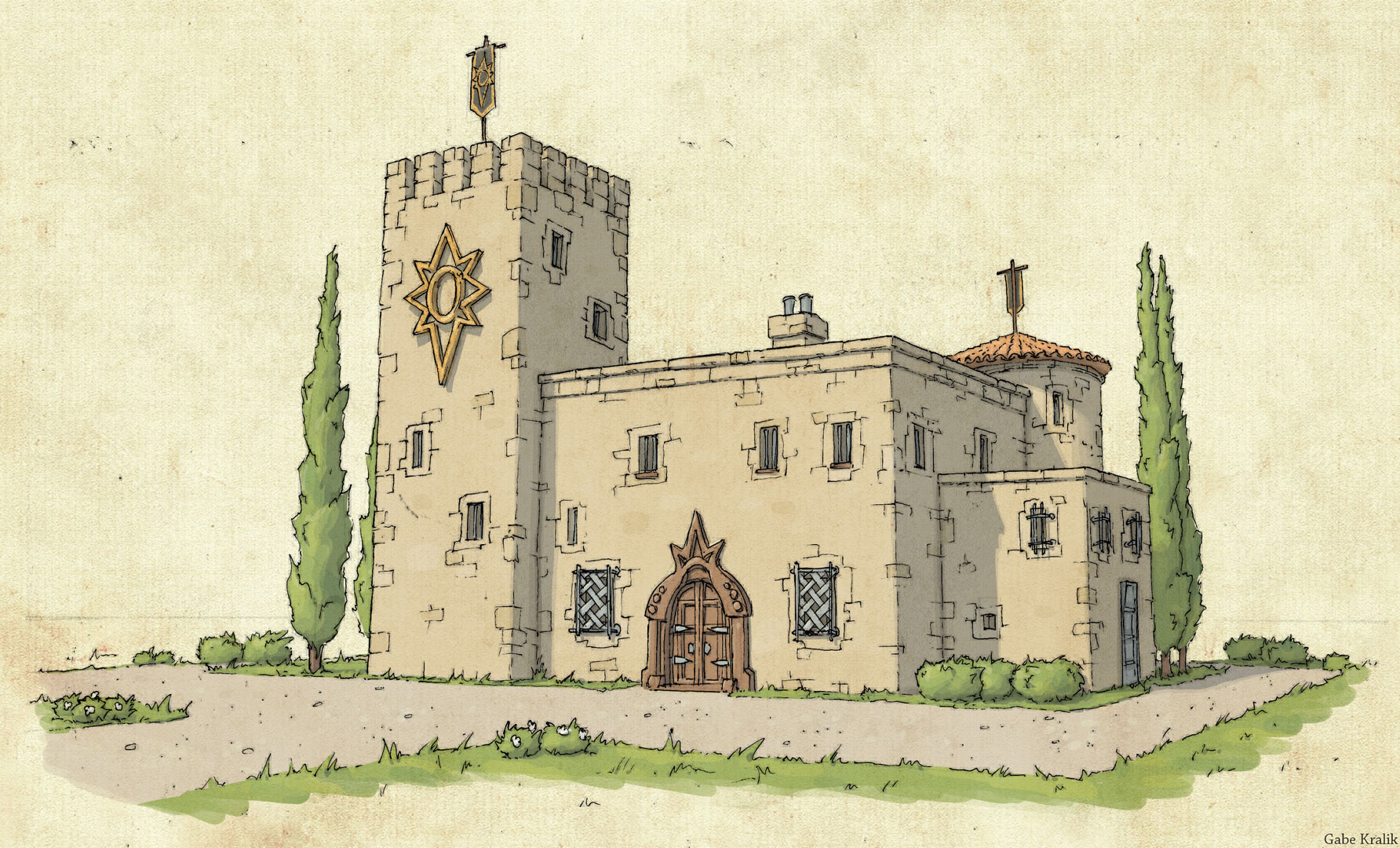The image depicts a detailed cartoon drawing of a two-story castle, front and center. The castle's square main body is constructed with stone and is yellow or beige in color. Prominent heavy wooden double doors dominate the center facade, flanked by two large windows at the bottom featuring crisscross patterns and barred smaller windows above. On the right, an additional section of the building with another door and similar windows is visible, with a shorter round tower situated behind it. To the left, a taller square tower reminiscent of castle architecture rises an additional story, featuring a flag with a star-shaped emblem at the top and an identical emblem on its facade. The entire structure is surrounded by a tan ground, with vibrant green grass, tall skinny trees, and bushes outlining a pathway in front of the castle. The artist's name, Gabe Craylake, is inscribed in the bottom right corner of the image.